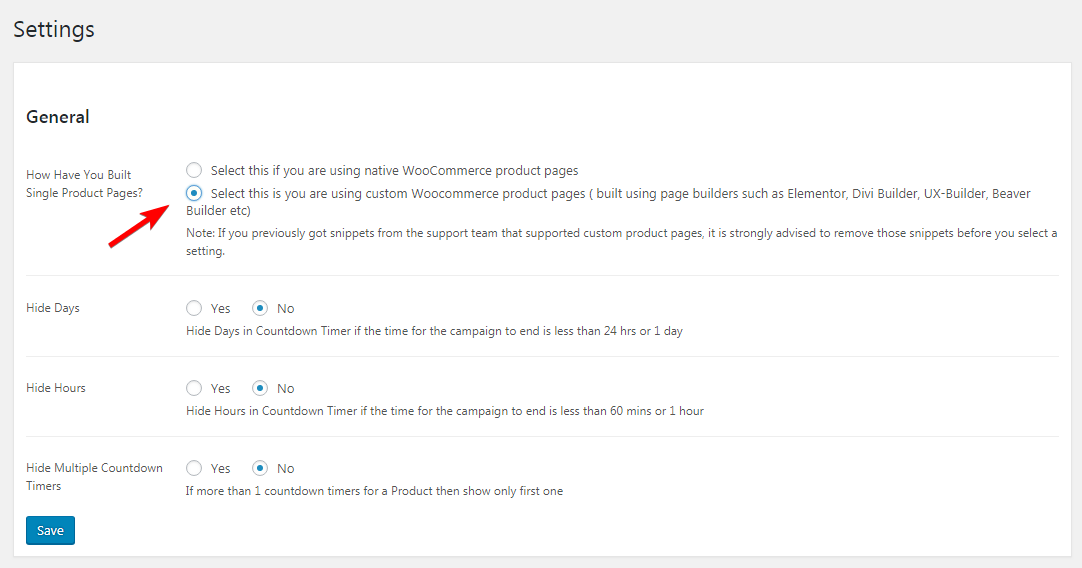The image depicts a settings page with a gray header labeled "Settings." The bulk of the page has a white background. On the left sidebar, the menu item "General" is highlighted.

The main section starts with a question, "How have you built single product pages?" Underneath are two selectable options. The first option consists of an unselected circle accompanied by the text, "Select this if you are using native WooCommerce product pages." 

The second option, which has a filled circle and a red arrow pointing to it, reads, "Select this if you are using custom WooCommerce product pages built using page builders such as Elementor, DiviBuilder, UXBuilder, BeaverBuilder, etc."

Below these options, there is a note advising users: "Note: If you previously got snippets from the support team that supported custom product pages, it is strongly advised to remove those snippets before you select a setting."

Following the note, the next section is labeled "Hide days," with two choices provided: "Yes" and "No." The circle next to "No" is filled in. The accompanying text states, "Hide days and countdown timer if the time for the campaign to end is less than 24 hours or one day."

Directly below, another section labeled "Hide hours" offers two choices, "Yes" and "No," with the circle next to "No" filled in. The associated text reads, "Hide hours and countdown timer if the time for the campaign to end is less than 60 minutes or one hour."

The next option, "Hide multiple countdown timers," also has "Yes" and "No" as choices, with the circle next to "No" filled in. The description states, "If more than one countdown timer is for a product, then show only the first one."

At the bottom of the page, a blue button labeled "Save" is present.